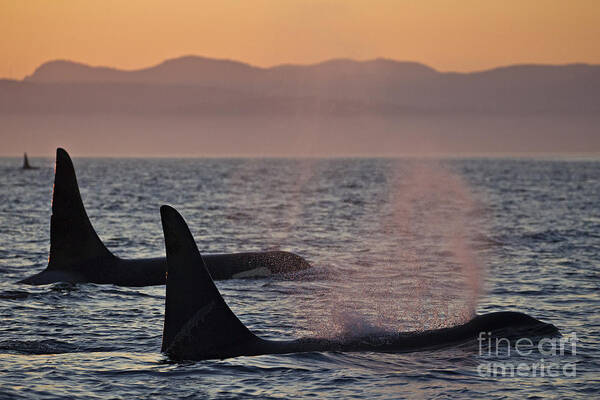The image captures a vivid, dynamic scene of the ocean at sunset, featuring three killer whales. In the foreground, two close-up whales, all black with striking dorsal fins, are surfacing, one of them spewing water from its blowhole, while in the background, a third whale's tail is visible. The water is a rich, dark blue, contrasting with the light orange-beige sky that casts a hazy, purple-gray film over distant mountain ranges. The entire setting is bathed in the soft, colorful light of the setting sun. The words "Fine Art America" are clearly visible in the bottom right corner, with "Fine" in thinner letters and "Art" and "America" in thicker, lowercase letters, complementing the overall aesthetic of the image.